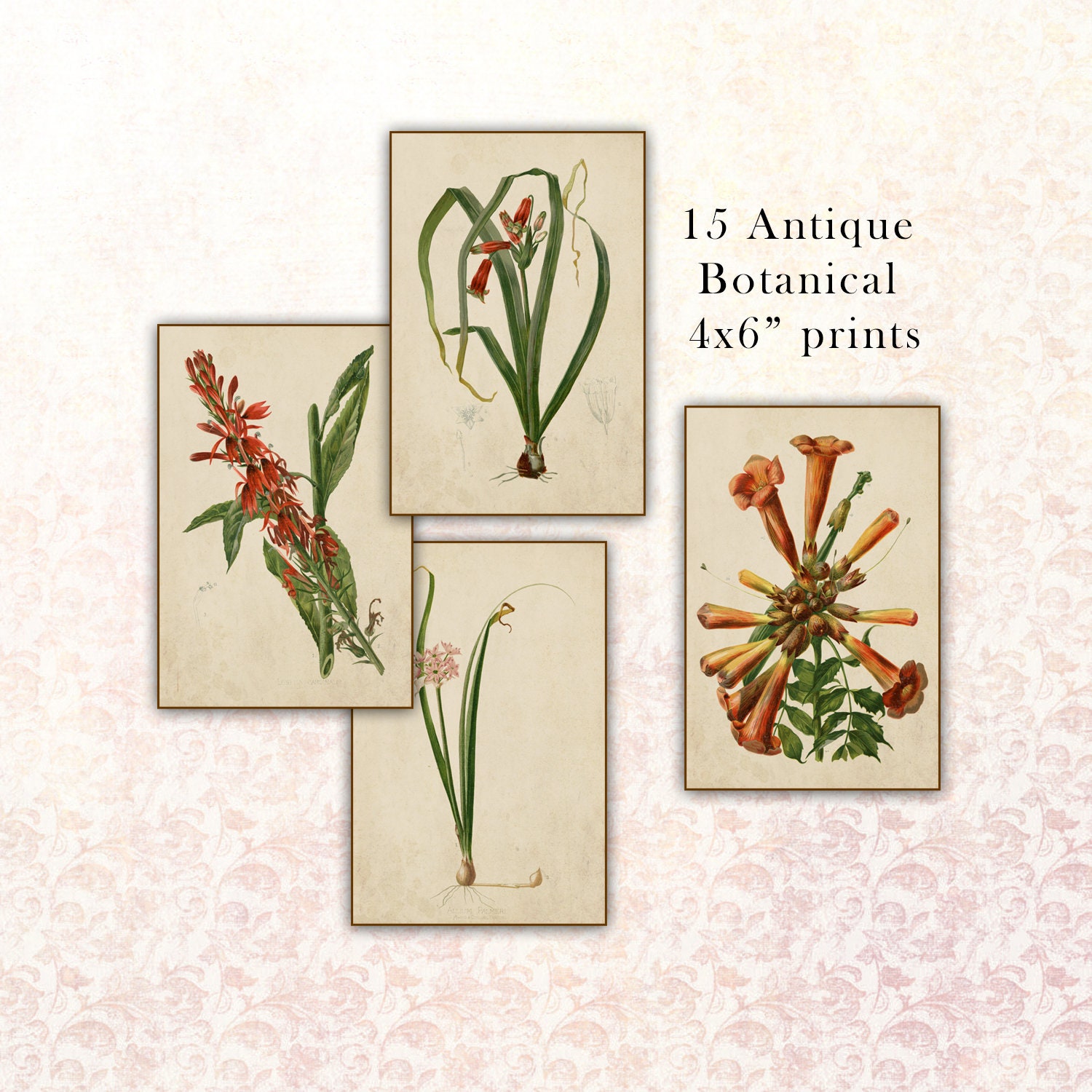The image is a full-color, vertically rectangular print piece with no border. The background features a subtle, white with light pink or light purple floral design, reminiscent of wallpaper. At the upper right, in black text, it reads "15 Antique Botanical 4x6 Prints." Displayed in the center are four vertically-oriented botanical prints, each showcasing different flowers. 

1. The print at the far right displays a tube-shaped flower with some bulbs not yet bloomed, accompanied by green leaves.
2. The print at the bottom highlights mostly green leaves with a small pink flower.
3. To the left, another print illustrates green leaves alongside a red flower.
4. The print at the top left showcases mostly leaves with small red flowers, some of which appear to be shriveled.

This collection offers a glimpse into antique botanical art, reflecting a delicate and detailed portrayal of various plants.